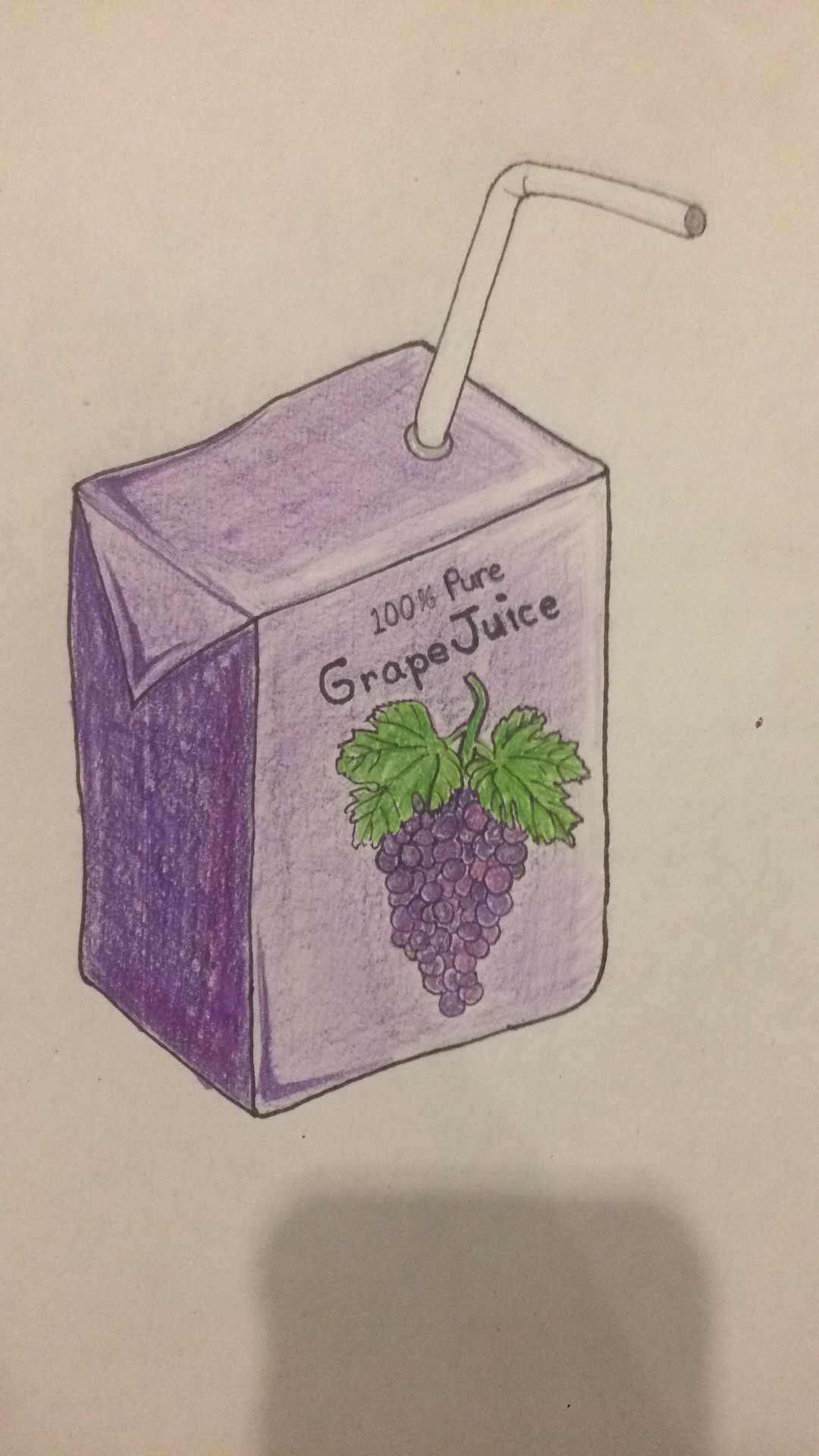The image is a colored pencil drawing of a rectangular grape juice carton on a white surface. The carton is predominantly purple, with the front and top sections depicted in lighter shades to create a three-dimensional effect. On the front, in black text, it reads "100% pure grape juice" above an illustration of blue grapes adorned with two green leaves and a green stem. A white straw, with a slight bend, is inserted into a hole at the top of the carton. The drawing also includes a grey shadow of the carton, giving it a more realistic touch. Additionally, at the bottom of the image, the shadow of a phone is visible, indicating that the artwork was photographed on drawing paper in portrait orientation.